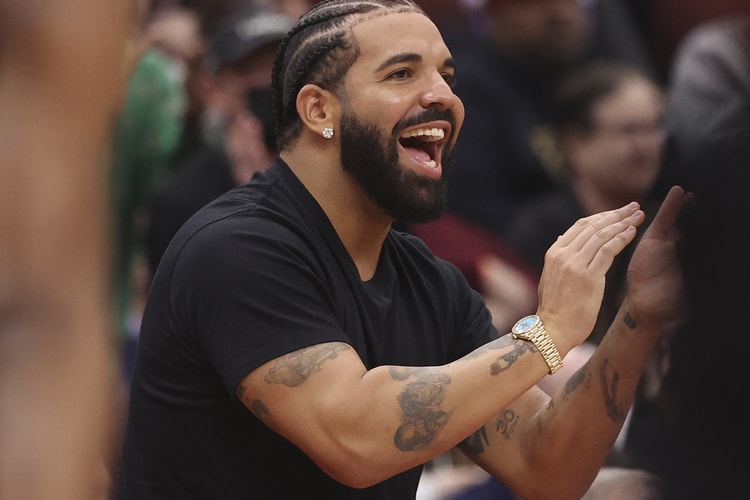In the center of the image, the famous musician Drake is prominently featured. He is a light-skinned black man with a muscular build, wearing a tight black t-shirt that highlights his physique. Drake is captured in a moment of joy, his mouth wide open in a huge smile, with his teeth and tongue visible. He seems to be in the midst of clapping his hands, indicating something has made him really happy. 

Drake's appearance is detailed and striking: he has a well-groomed black beard and his hair is styled in tight braids or cornrows. His arms are adorned with various black tattoos, including a tattoo of the number 30 on one of his arms. He accessorizes with diamond-studded earrings and a gold wristwatch on his right wrist. 

The background of the image is intentionally blurred, creating a sharp focus on Drake. The blurred backdrop reveals shades of brown on the left and a crowd of indistinct people on the right, suggesting a lively atmosphere. The people seem to be dressed in darker clothing and appear to be seated, all looking in the same direction as Drake, contributing to the dynamic and joyful mood of the scene.